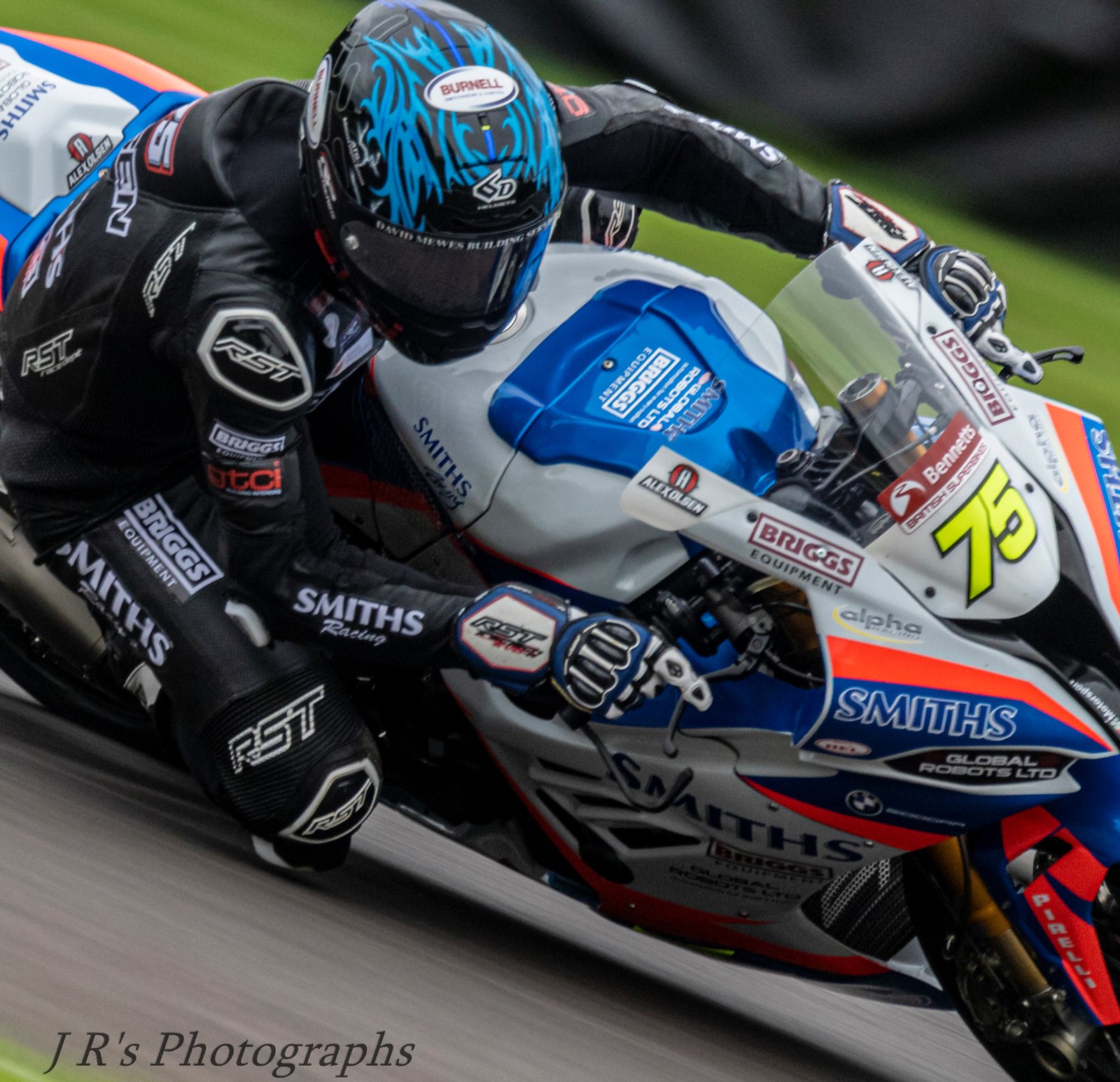The image captures a dynamic scene of a biker aggressively leaning into a turn on a sleek, compact motorcycle designed for racing. The motorcycle, presented in a blend of gray with dark blue and bright orange trim, is prominently numbered 75 in bold, bright yellow on its partially visible front end to the right of the image. The rider, centered towards the left of the photograph, is donned in a predominantly black racing suit adorned with numerous logos including R.S.T., Smiths, Briggs, and Bernal, matching the logos scattered across the bike's body as well. His helmet, featuring a blue flame pattern, complements the blue accents on the bike. Despite the motion blur, the gray asphalt is discernible beneath the rider, while a field of green grass in the upper background and a black track wall reinforce the high-speed nature of the moment. The dramatic lean brings the motorcycle perilously close to the ground, indicating a left turn, with the rider's knee and feet almost skimming the track. The scene is marked at the bottom left corner with a watermark reading "JR's Photographs" in black font.